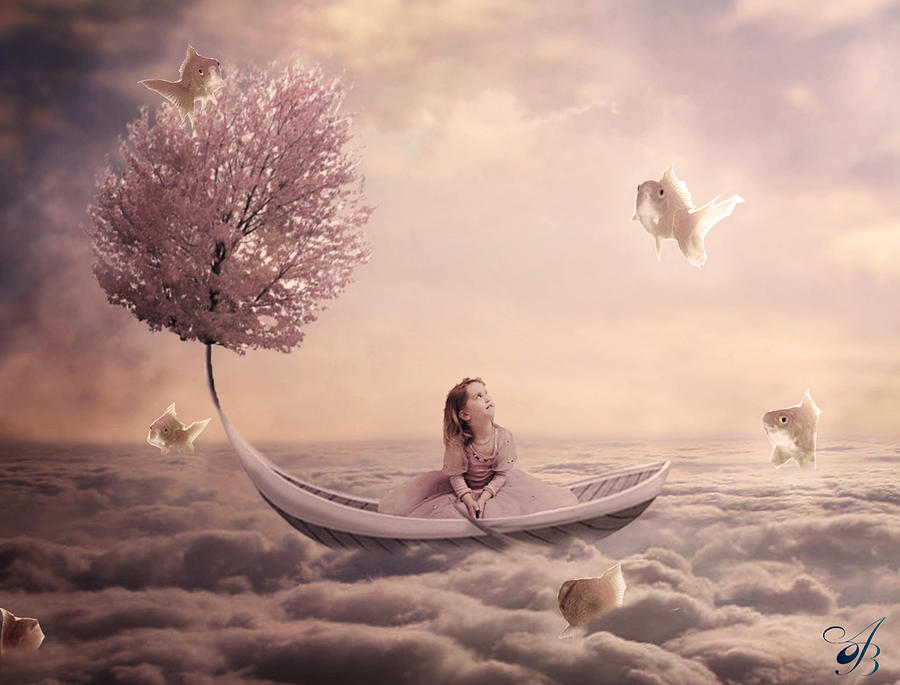In this whimsical, dream-like image with a predominantly pinkish hue, a young girl in a pink dress sits in the middle of a delicate boat resembling a large leaf. The boat appears to float atop a bed of fluffy clouds, accompanied by a cherry blossom tree with vivid pink blooms on the left, which serves almost like a sail. She gazes upwards with a look of wonder at several floating fish around her—a total of five fish can be seen, with some appearing to swim through the air while others hover beside her ethereal vessel. In the distant background, there are subtle hints that resemble water, adding to the surreal, fantastical nature of this scene. The bottom right corner bears a cursive watermark with the initials "AB."